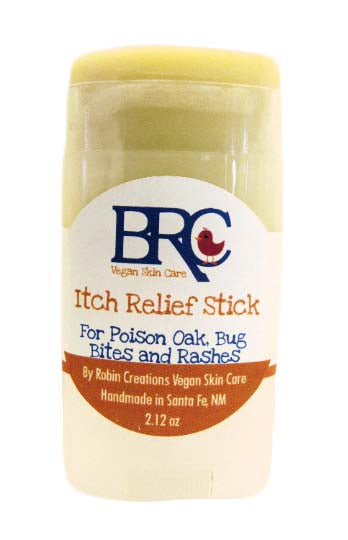The image depicts a 2.12 oz Itch Relief Stick from BRC Vegan Skin Care, specifically for treating poison oak, bug bites, and rashes. The product is handmade in Santa Fe, New Mexico, by Robin Creations Vegan Skin Care. The stick, which resembles a deodorant stick, has a cream-colored (light yellow) waxy appearance and is housed in a plastic container with a solid ivory-white base and a clear upper section. The product label features the brand's logo, "BRC," in capital navy blue letters accompanied by a red bird logo with an orange beak and legs. The label is white and circular, detailing the product name and usage instructions. The photograph is taken against a seamless, solid white background, creating the impression that the product is floating in a void, directing full attention to the product itself. The lid of the container is not present in the image, and the stick is exposed, emphasizing the product's texture and color.